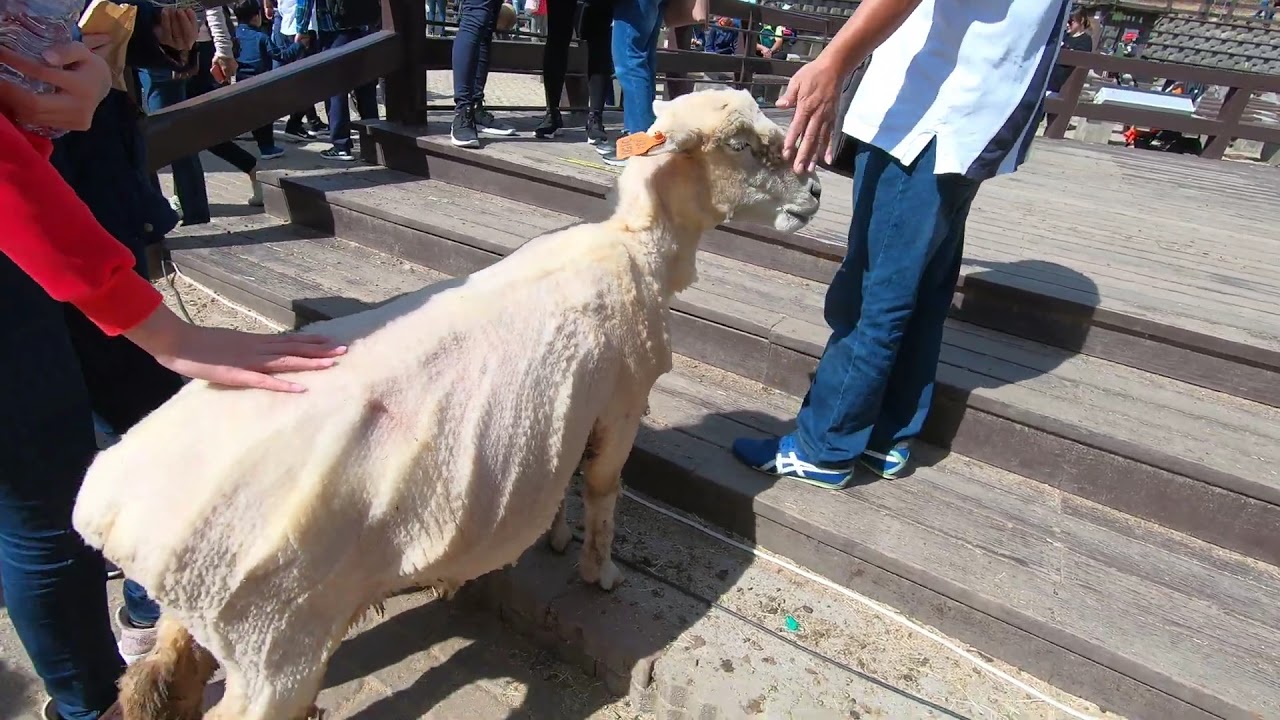In this horizontally aligned rectangular picture taken outdoors, there is a goat prominently placed from the middle to the left side of the image. The goat, which sports a freshly shaven, somewhat awkward appearance, is covered with a beige blanket and bears an orange tag on its right ear. Its back legs are positioned at the bottom of a small wooden staircase, while its front legs are a few steps up, leading towards a wooden deck area. A male figure, visible only from the waist down, stands on a step in front of the goat, wearing jeans, blue and white tennis shoes, and a light-colored short-sleeved shirt with a vented hem. He is gently petting the goat's face with his left hand. To the left, another individual, identifiable by their blue jeans and long-sleeved red shirt, has their hand placed on the goat's back. In the background, several other people are partially visible, mostly by their legs and feet, gathered around the wooden deck area behind a wooden fence, contributing to a petting zoo-like atmosphere.